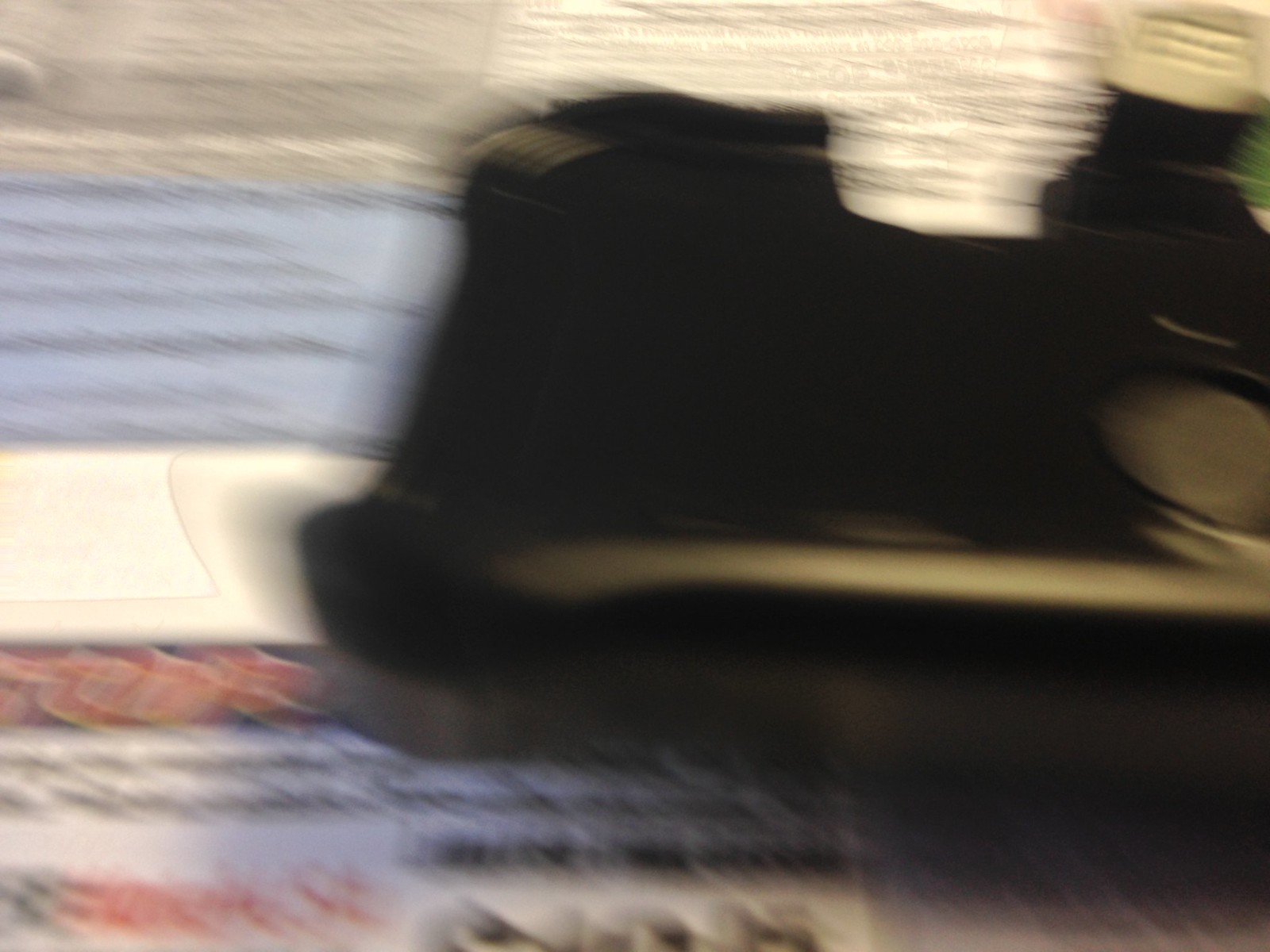A very blurry close-up photograph captures an indistinct black, plastic object that appears to be square-shaped with rounded edges, possibly a phone case, positioned atop a surface displaying scattered text and colored rectangles. The background, likely a newspaper or flyer, shows hints of black text at the top center and a small blue rectangle to the left. The overall image is unfocused, making it difficult to clearly identify details or the exact nature of the scene.